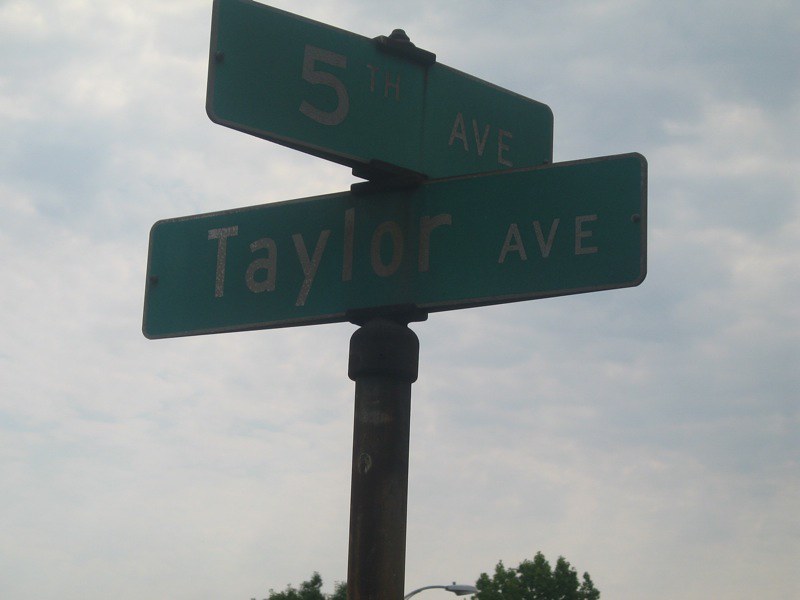This is a photograph taken during the daytime, capturing a street scene. The background features a pastel light blue sky filled with fluffy, white clouds, creating a soft and serene atmosphere. Near the bottom of the image, we discern the tops of two trees with green leaves, flanking a street lamp that is mounted on the same pole as the signs. The central focus is a cylindrical gray pole rising from the bottom of the frame, which looks somewhat dirty and weathered but not rusted.

Attached to the pole are two slightly faded green rectangular street signs with white text. The top sign reads "5th Avenue," while the longer bottom sign reads "Taylor Avenue." The signs are not perfectly aligned; instead, they are tilted at angles, creating a crisscrossed arrangement. The street lamp and the tips of the trees complete this urban visual vignette against a sky dominated by plentiful clouds.